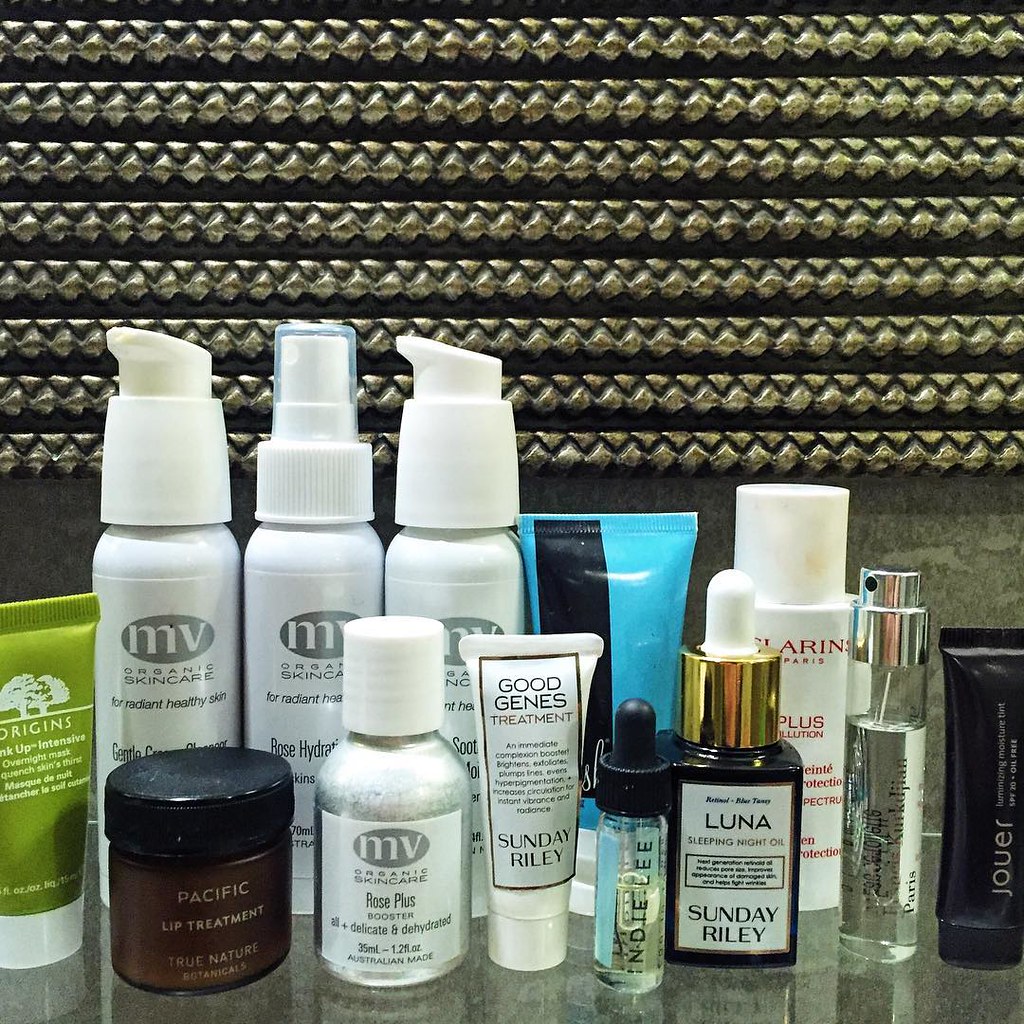This is a vibrant and detailed composition of various beauty products meticulously arranged on a tabletop. Featured prominently in the group is a green bottle from Origins, though its specific contents are not visible. In the lineup, there are three taller bottles displaying the logo "MV" and marked as Organic Skin Care products, promoting Radiant Healthy Skin. One of these MV bottles appears to be a rose hydrating product, though the full titles are obscured. Also in the arrangement is a striking blue bottle, juxtaposed against a Clarins bottle prominently placed towards the front. Among the collection is a Pacific Lip Treatment by True Nature Botanicals, an MV Organic Skin Care Rose Plus Booster, and a Good Genes Treatment by Sunday Riley. Adding to the array, there's a bottle of an unidentified liquid, followed by Luna Sleeping Night Oil by Sunday Riley, another unidentified bottle, and lastly, a Jour bottle. Each product in this sophisticated collection exudes an air of luxury and efficacy, catering to various skincare needs.